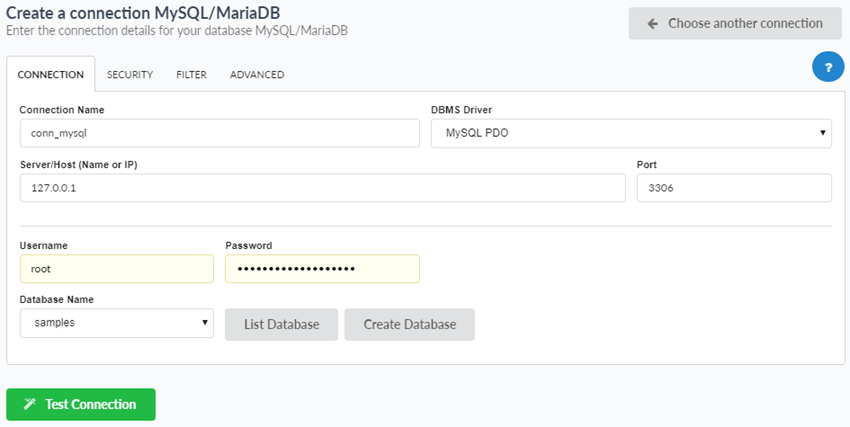The screenshot depicts a user interface for creating a connection for MySQL or MariaDB databases. At the top, a title reads "Create a Connection for MySQL/MariaDB." Beneath it, in smaller text, it prompts the user to "Enter the connection details for your database: MySQL/MariaDB." 

On the right side, there's a gray box with an arrow pointing to the left, labeled "Choose another connection." Below this gray box is a blue circle with a question mark inside, indicating help or further information is available.

The interface has several tabs: "Connections," "Security," "Filter," and "Advance." The current tab selected is "Connection."

Within the "Connection" tab:
- The first input field is labeled "Connection Name," containing the pre-filled text "conn_mysql."
- The next field, a dropdown menu for the DBMS driver, has "MySQL PDO" selected.
- The "Server/Host" field, annotated with "name or IP," contains "127.0.0.1."
- The "Port" field is populated with "3306."
- Below these, two fields labeled "Username" and "Password" display "root" and black dots respectively, indicating a concealed password. Both fields have a pale yellow background.
- A dropdown menu for "Database Name" lists "samples" as the selected option.

At the bottom are two gray buttons labeled "List Database" and "Create Database." There is also a prominent green button with white text that says "Test Connection."

The entire layout of the input fields and buttons is designed to facilitate the process of establishing a MySQL/MariaDB database connection, guiding the user through each required detail step-by-step.